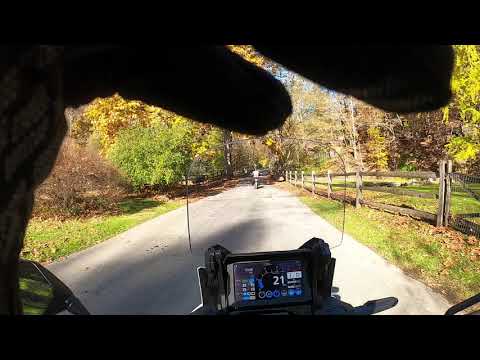This vivid color photograph captures a bright, sunny day from the perspective of someone riding a motorbike or scooter. The image, which appears to be taken with a GoPro camera mounted on the rider's helmet, looks out over the scooter’s windshield onto a gray paved road flanked by lush greenery. The road is lined with a small wooden fence on the right, and both sides of the path are bordered by grassy fields and clusters of trees. The trees are beginning to show signs of fall, displaying a mix of green, yellow, and brown leaves. Sunlight filters through the trees, casting reflections onto the road. In the foreground, just to the right of center at the bottom, a small black dashboard screen prominently displays the number "21" in white—possibly indicating the speed of the vehicle. The rider's left hand, visible as a black silhouette, is in front of the visor. Horizontally, the photograph is narrower than the black background that frames it, creating strips of black along the top and bottom of the image. To the left of the view, the edge of a rearview mirror is visible. Ahead, another rider on a bike or motorcycle can be seen, leading the way down this serene path.